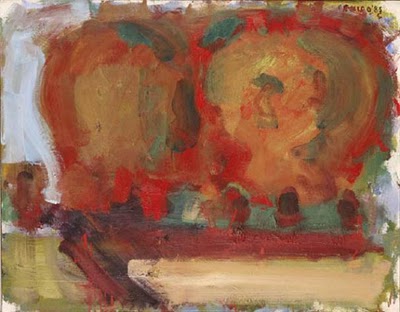The image in question appears to be an abstract oil painting, roughly two and a half inches high by three inches wide, with a near-square shape. Dominated by bold and smudged color patches, the composition features a beige horizontal smudge on the bottom right side, with a red smudge marking above it. In the lower left corner, there is a green smudge. The main focal point of the image is two large, messy, orange-yellow circles with green smudges, surrounded by darker orange hues, occupying the central portion of the painting. This section also integrates some tealish blue streaks. The background itself is a lighter blue, but with the various colors smudged into it, lending a textured, layered appearance.

The bottom edge of the painting showcases a distinctive light brown bar, overlaid with red and reddish-black strokes, creating a horizontal and diagonal motif. Above these, there are additional red and orange colored rings, layered with chunky red markings, sitting atop a maroon base, which in turn rests on a cream-colored foundation. Off to the very left, some white strokes run vertically upwards.

In the upper right corner, a signature rendered in dark red is visible, although it's illegible due to the language and indistinct letter formation.

With its blend of colors and forms, the painting's exact subject remains elusive, though interpretations vary from abstract atmospheric depictions to possible representations of objects like boats or apples.